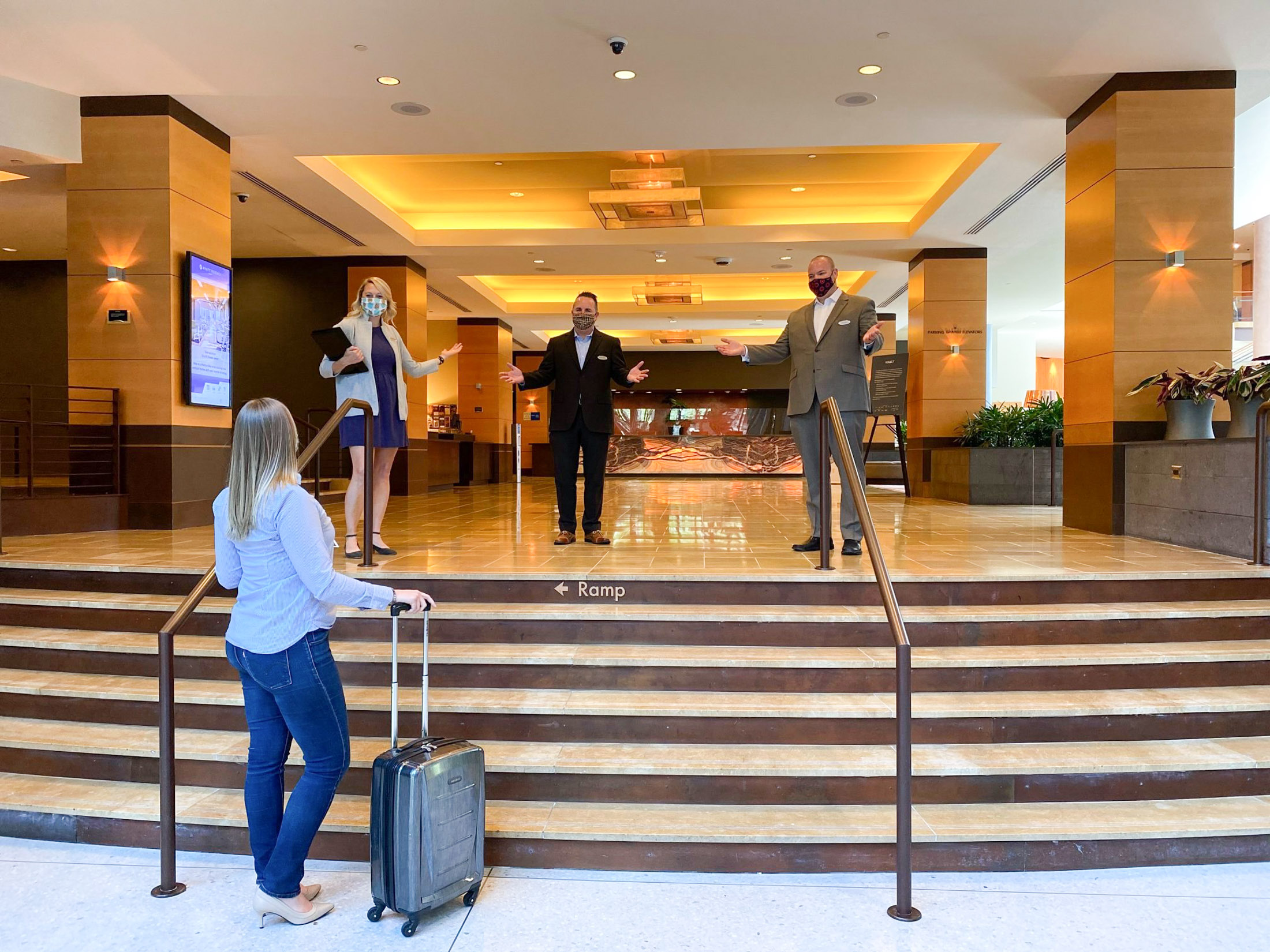The image portrays a well-lit, modern indoor setting that appears to be a hotel lobby or mall entrance. The lobby features a staircase with bronze-colored railings and six light brown steps with dark brown interstitial accents. The ceiling is white with built-in lights and square golden areas housing chandeliers. Light tan columns with dark brown bases flank the sides of the image, adorned with planter boxes containing green plants, and there's a mural visible in the far background.

At the top of the stairs stand three individuals, all wearing face masks. On the left, a blonde woman in a blue mid-thigh dress paired with a light gray sweater holds a black square object, possibly a clipboard, and extends her hand in a welcoming gesture. Next to her, a man in a dark suit with a light-colored undershirt and brown shoes also stretches out his arms in greeting. On the right, another man dressed in a light brown suit, white or blue shirt, and brown shoes similarly extends his arms. 

At the bottom of the stairs stands a woman wearing a light blue top, dark blue jeans, and white or gray high heels. She holds a silver, wheeled suitcase with a handle in her right hand and looks upwards toward the welcoming trio above. The general ambiance is inviting, emphasized by the pristine, shiny tiled floor and the elegant design elements throughout the space.